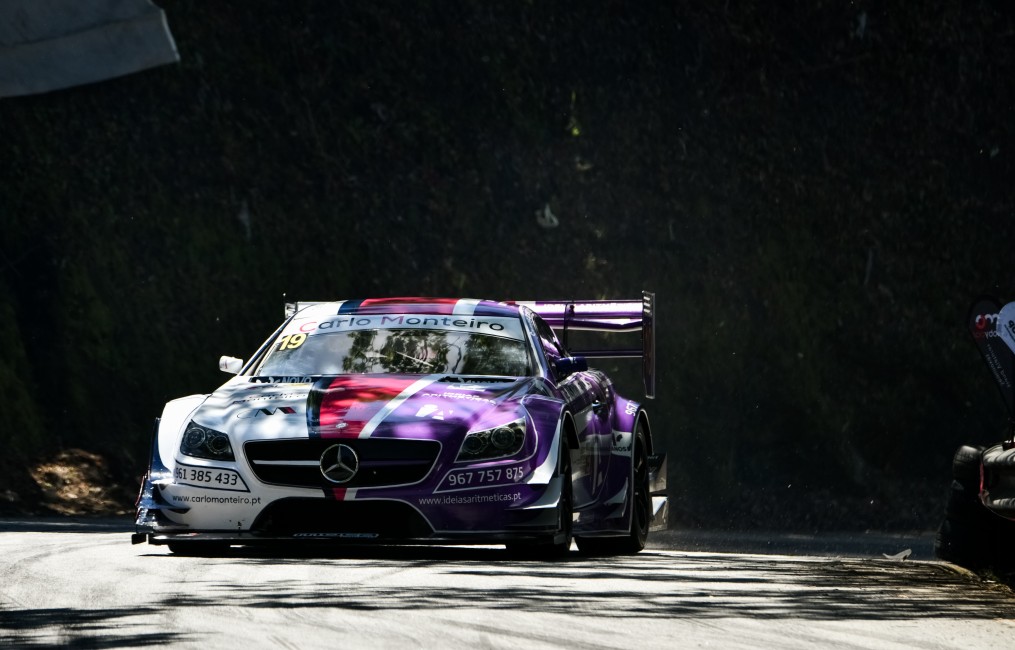This outdoor photograph captures a striking image of a highly modified Mercedes-Benz race car, possibly during a test drive in a tree-lined mountainous area. The car, prominently positioned on a paved road, features a unique and vibrant color scheme: the left side is white, transitioning to red in the middle accented with black and white stripes, and then to purple on the right side. The car boasts a massive rear wing and a flared-out fender for wider wheels, indicating its high-performance capabilities. 

Prominently displayed across the top of the windshield is the name “Carlo Monteiro” in black lettering on a white banner, a key identifier for the vehicle. There is also a distinct yellow number “19” set against a small black box on the car's left side. Additionally, various logos and numbers like "561385433" and "967757875" are seen adorning the front, further emphasizing its race-ready aesthetics. The blurred green trees in the background provide a dynamic contrast to the car's details, making it the undeniable focal point of this high-intensity photograph.